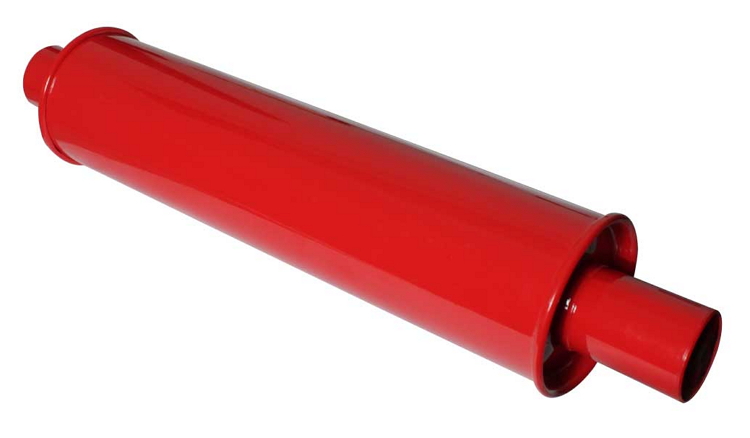This photograph showcases a glossy red cylindrical object, reminiscent of a muffler or a rolling pin. The material appears to be either metal or plastic, with a highly reflective, glossy surface. The object features a prominent wide middle section that tapers drastically at both ends into smaller diameter pipes. The entire structure is clearly hollow, and the smaller ends extend out from the main cylinder by a few inches, suggesting a design where these sections are meant to be handled or connected. The object is set against a transparent background and is depicted at a diagonal angle, highlighting its shiny surface and intricate shape.